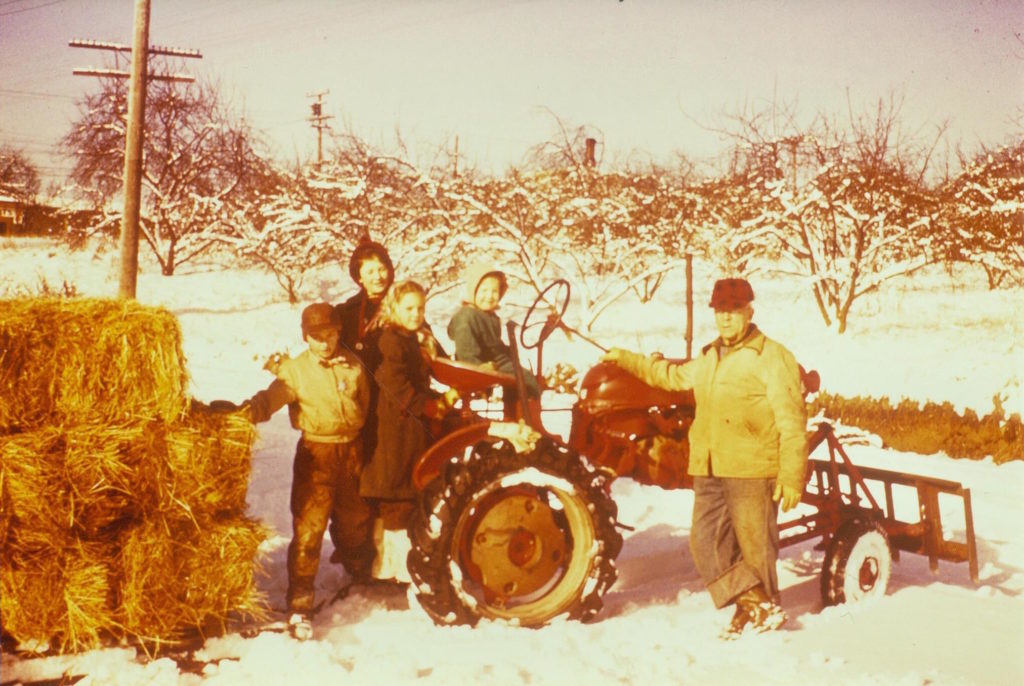A horizontally oriented, vintage color slide captures a nostalgic winter family portrait, tinged with the golden hue of age that has faded much of the original cyan. The scene centers around a cheerful family standing amidst the snow, fully dressed in winter boots and gear. At the heart of this tableau is a weathered red tractor, presumably the focal point of the family's agrarian lifestyle. 

To the left, a mound of hay sits quietly under the soft shadows cast by a low row of trees and a solitary telephone pole in the distance. The familial warmth contrasts the cold surroundings as they gather around the tractor. A child perches delightedly on the tractor seat, while three others cluster behind them. The mother stands protectively behind her children, encapsulating the essence of familial unity. 

The father exudes a rugged, hardworking charm in his lumberjack jacket and rolled-up blue jeans, his right hand resolutely gripping the tractor wheel. Their smiles, directed towards the camera, convey a timeless sense of joy and togetherness, perfectly preserved in this aged yet treasured slide.